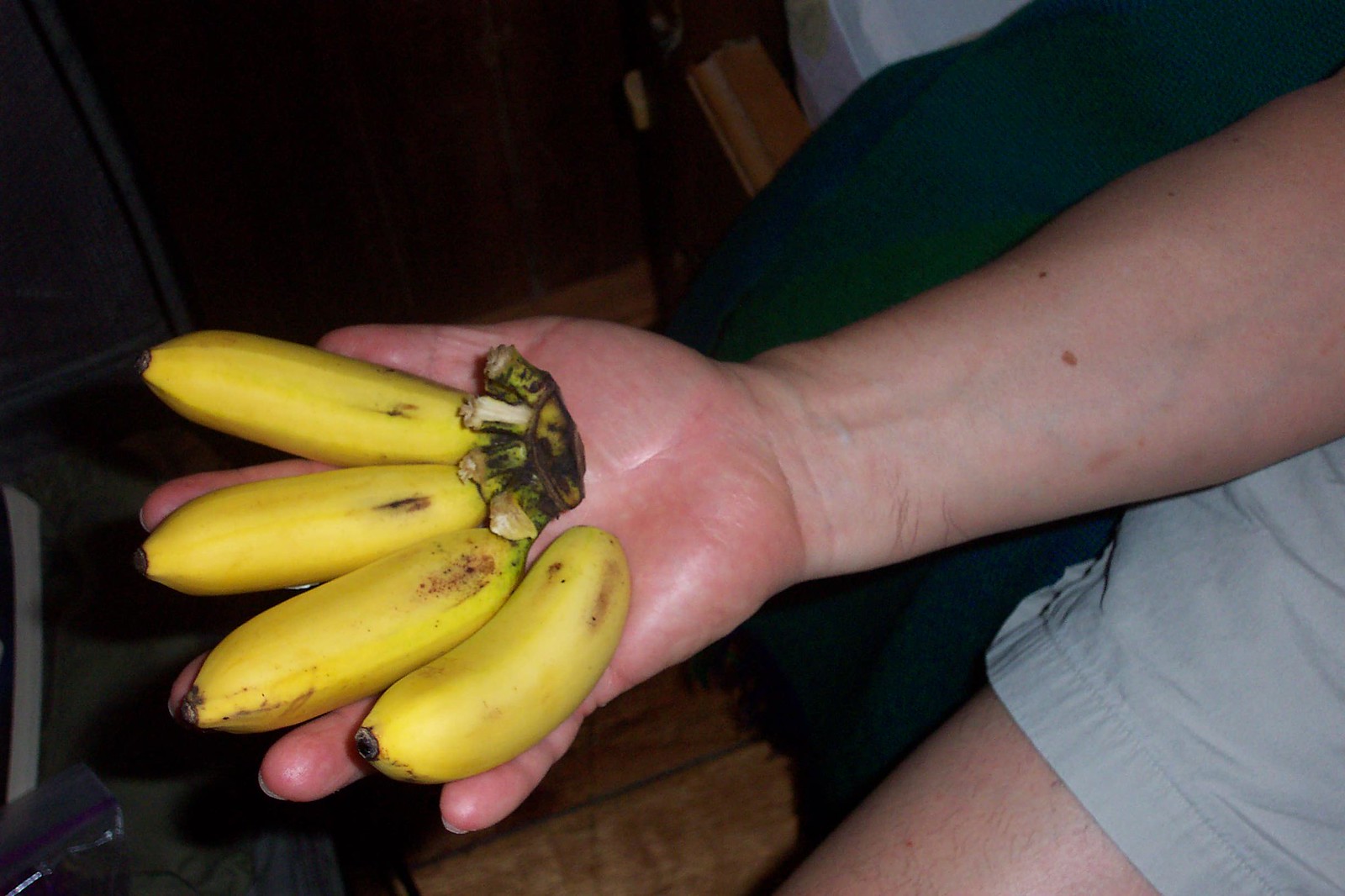A person is sitting with their arm resting on the black cushioned armrest of a chair. The image is focused on their forearm and hand, which is palm-up and holding four small, yellow Saba bananas. Three bananas are still attached to the stem, while the fourth is separated. These ripe bananas feature some brown spots and a brown circular mark at the bottom, with hints of green near the stem. The background includes a brown wooden floor and some black elements, with a patch of gray visible on the left side.